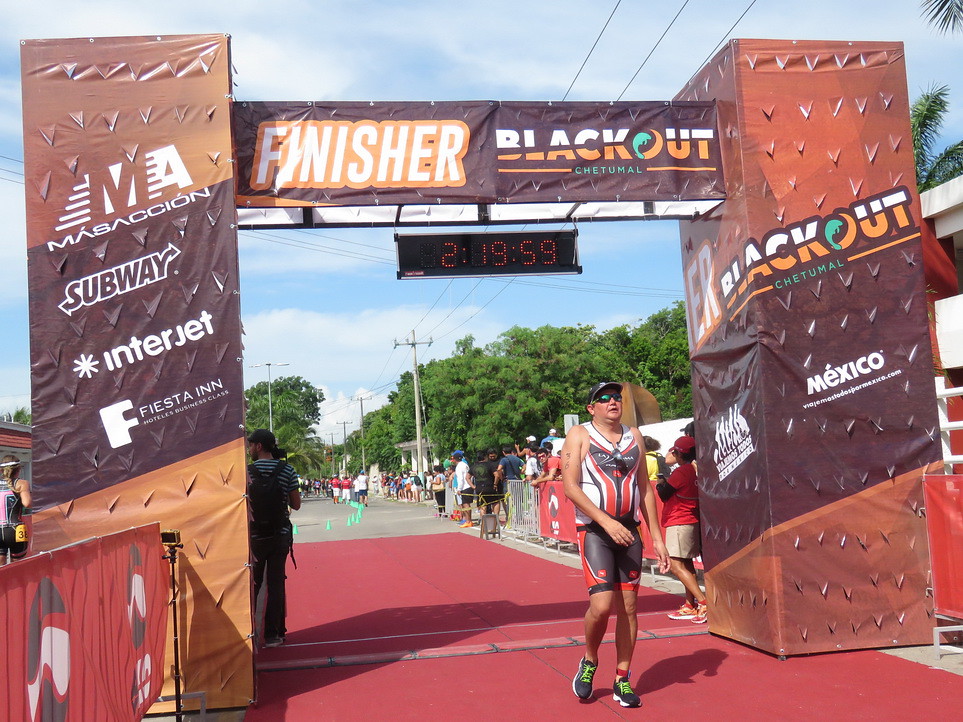This detailed photograph captures the finish line of a marathon race held outdoors during the middle of the day, under a clear blue sky with white clouds. The finish line is prominently positioned at the center of the image, marked by two tall pillars and a crossbeam adorned with numerous sponsor logos, including Subway, Interjet, Fiesta Inn, and SSE. A digital clock hanging from the crossbeam displays the time 2:19:59. The horizontal part of the finish line structure prominently displays the words "Finisher, Blackout, Chetumal."

In the foreground, a male runner, wearing black shorts, dark sneakers with green laces, and a sleeveless white top, is seen crossing the finish line. He appears exhausted, donning a hat, sunglasses, and a second pair of sunglasses affixed to the top of his shirt. The number 36, presumably his runner's number, is visible on his arm. Beneath him lies a red carpet that stretches along the race path.

On either side of the racecourse, barriers confine the route, lined with spectators cheering behind them. The scene is lively, with people, possibly including camera crews and officials, visible in the background. The setting is detailed with trees, light posts, and telephone poles flanking the sides, adding to the vibrant atmosphere of the event.